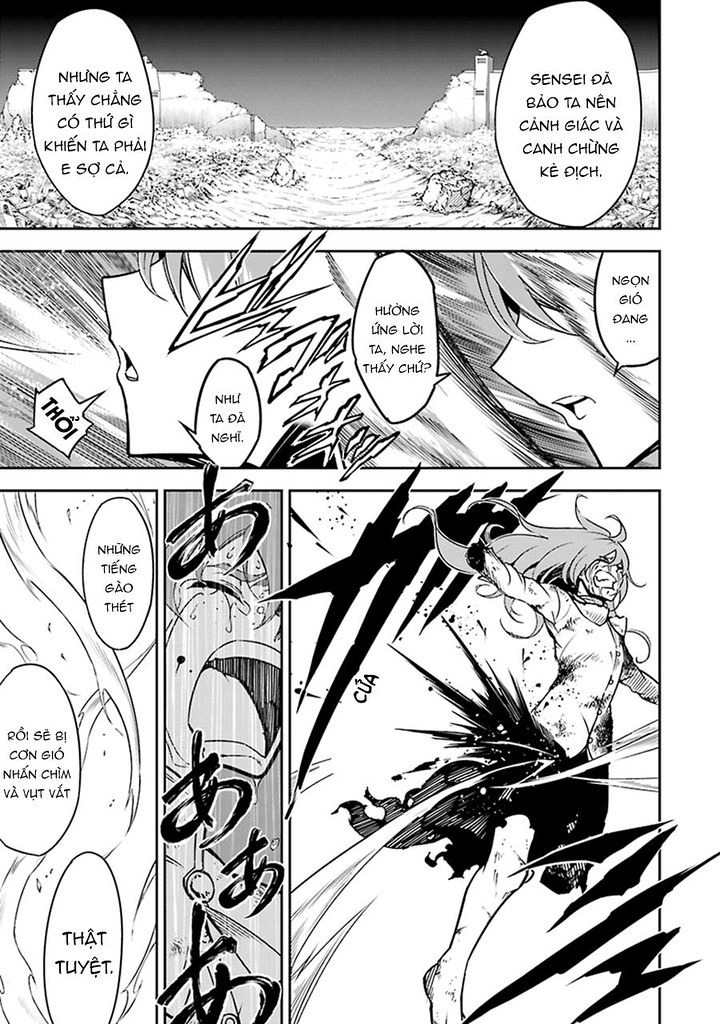This image features a black and white manga page composed of several illustrated panels, each containing word bubbles with an oriental script, likely Southeast Asian. The first panel depicts an animated dirt road flanked by grassy patches. In this scene, there are two speech bubbles with foreign text. Following this, the next panel continues in black and white with a different design and contains four distinct word bubbles filled with the same foreign language. The subsequent two panels are laid out vertically, side by side, and feature a total of three word balloons.

In the final panel, a lone character with long hair is depicted amidst dynamic, lightning-like streaks of energy. This character, dressed in a white top and black skirt or shorts, is striking a powerful stance, reminiscent of a martial arts pose, indicating a display of superhuman abilities. There are no other characters or weapons present, centering all attention on this singular, ancient-world superhero figure.